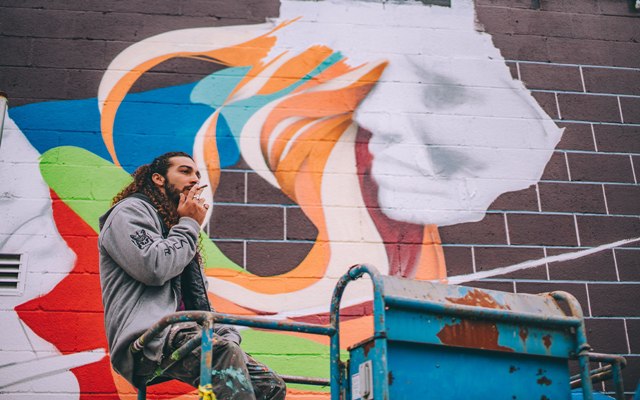In the photograph, a young man with long, frizzy, curly brown hair and a beard is sitting on the edge of a worn, blue metal hoist lift, which shows significant rust and peeling paint. He is dressed in a gray long-sleeve hoodie and paint-splattered pants, indicating he might be the artist working on the mural behind him. The man is relaxed, smoking a cigarette with his right hand, which also sports two rings. He gazes into the distance towards the right. The background features a dark red brick wall, some sections outlined with white mortar, prominently displaying a graffiti art piece. The mural depicts a woman's face in white, with her hair transforming into vibrant swirls of oranges, pinks, blues, and whites. To the left of her face appears the outline of another person, also in white, enhancing the artistic and dynamic ambiance of the scene.